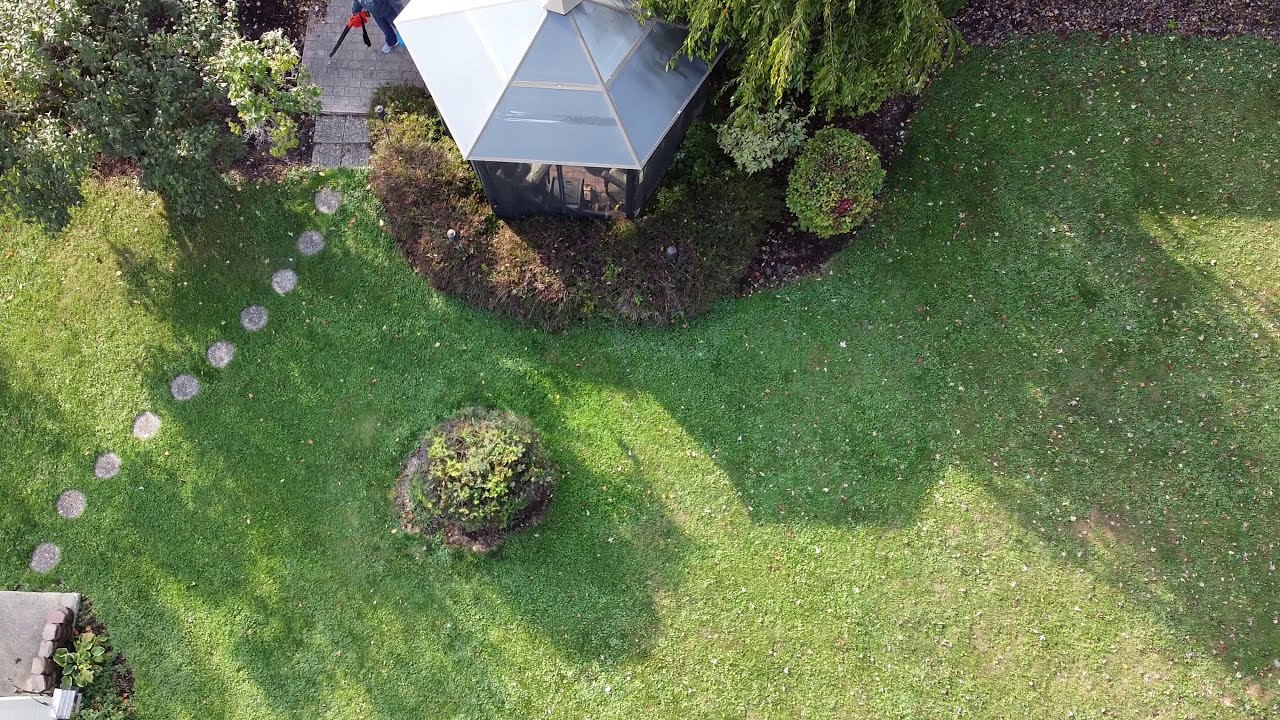This aerial image captures a meticulously maintained garden, likely someone's backyard. The central focus is a lush, medium-green lawn dotted with what appear to be scattered white dandelion seeds or possibly petals. In the lower left corner, a small cement patio introduces a series of approximately ten round, gray stepping stones that form a path across the grass, leading to another stone patio at the top. Adjacent to this initial patio, a hosta plant adds greenery, while a person, possibly using a red and black leaf blower, is visible on the upper left patio.

Dominating the right-center of the image is a hexagonal gazebo with a light gray or light blue metal roof, surrounded by low bushes, medium trees, and some shrubbery. The sides of the gazebo are covered with either mesh netting or glass. Towards the center of the yard, a circular arrangement of flowering bushes adds a touch of color, and the entire scene is bathed in sunlight, casting shadows from the structures and foliage across the scene, from the upper left to the lower right. This picturesque and well-kept garden area evokes a sense of tranquility and order.